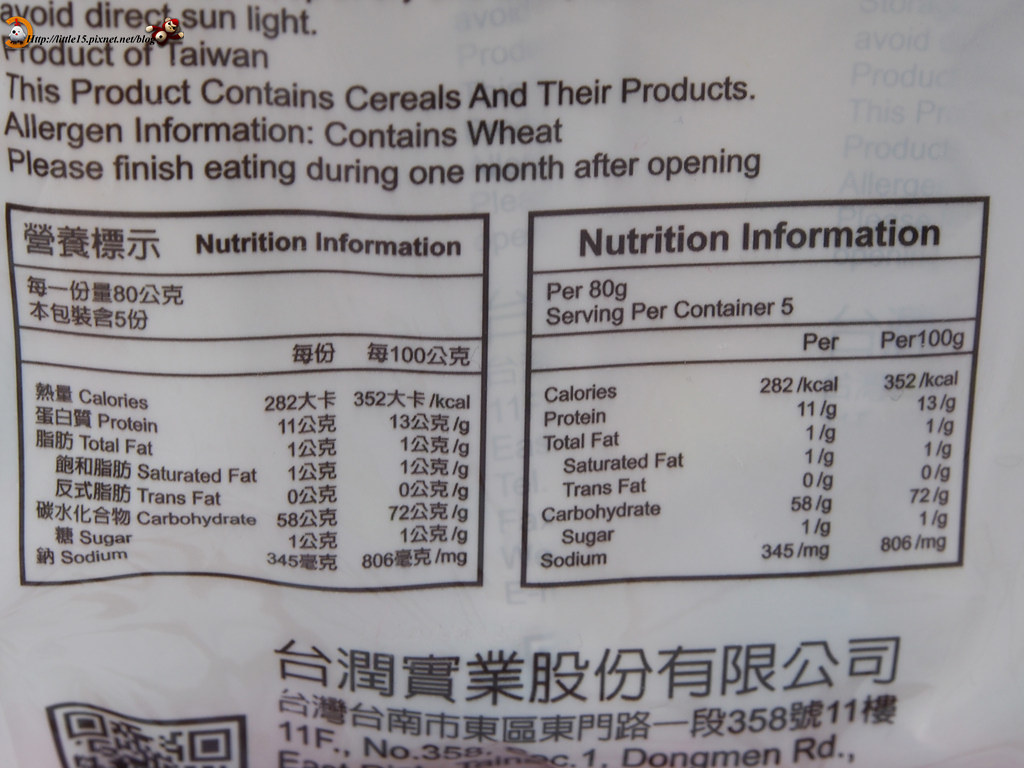This is a photograph of a product label with a white background. At the top of the image, on one side, there is a small cartoon icon in white with an orange section over it, next to a very small website address in black. To the right of this address, a red monkey-like figure is visible. The top section of the label contains a nutrient label and several important notices in black text. Starting from the top left, it reads: "Avoid direct sunlight," followed by "Product of Taiwan," and then "This product contains cereals and their products." The allergen information indicates that the product "contains wheat." Instructions state, "Please finish eating during one month after opening." Below these notices, there are two square panels side by side, outlined in black, that list the nutritional information. The panel on the right is labeled "Nutrition Information" in bold black text, with detailed nutrition facts listed below. The panel on the left contains four Chinese characters in the upper left corner, alongside more nutritional details and additional lines of Chinese characters. In the lower left corner of this panel, a QR code can be seen alongside more character symbols.